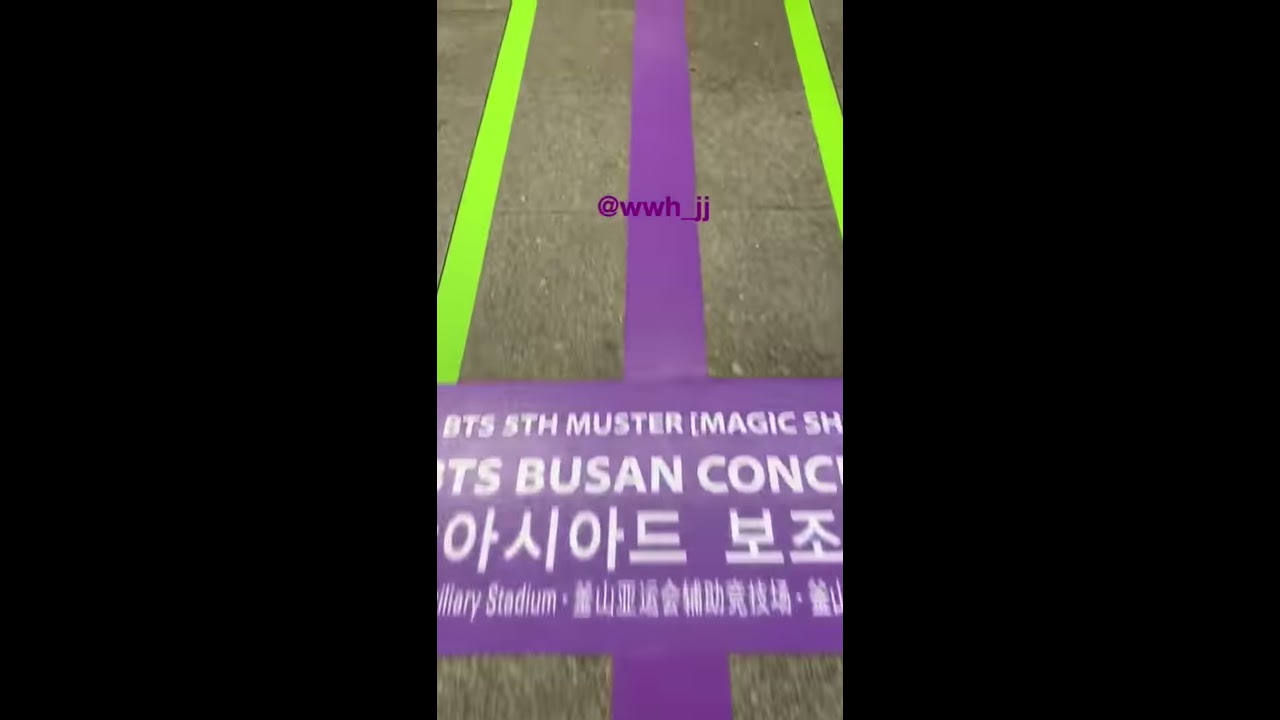The image is a vertical photo that occupies the central strip of the frame, flanked by large black rectangles on either side, creating a narrow, focused view. The central picture appears to depict a section of a pavement or sidewalk, marked by a prominent purple line running vertically down its center. On either side of this purple line, there are neon green or greenish-yellow stripes outlining the edges. Near the base of the image, overlapping the purple line and extending to the green boundaries, is a large purple rectangle containing white text. This text reads "BTS 5th Muster Magic Show" followed by "Busan" and some Korean characters. Additionally, there is an at-sign username located above the purple rectangle in the middle of the image, displayed as "@WWH_JJ." The overall composition suggests an advertisement or sign, possibly related to an event in Busan, Korea.